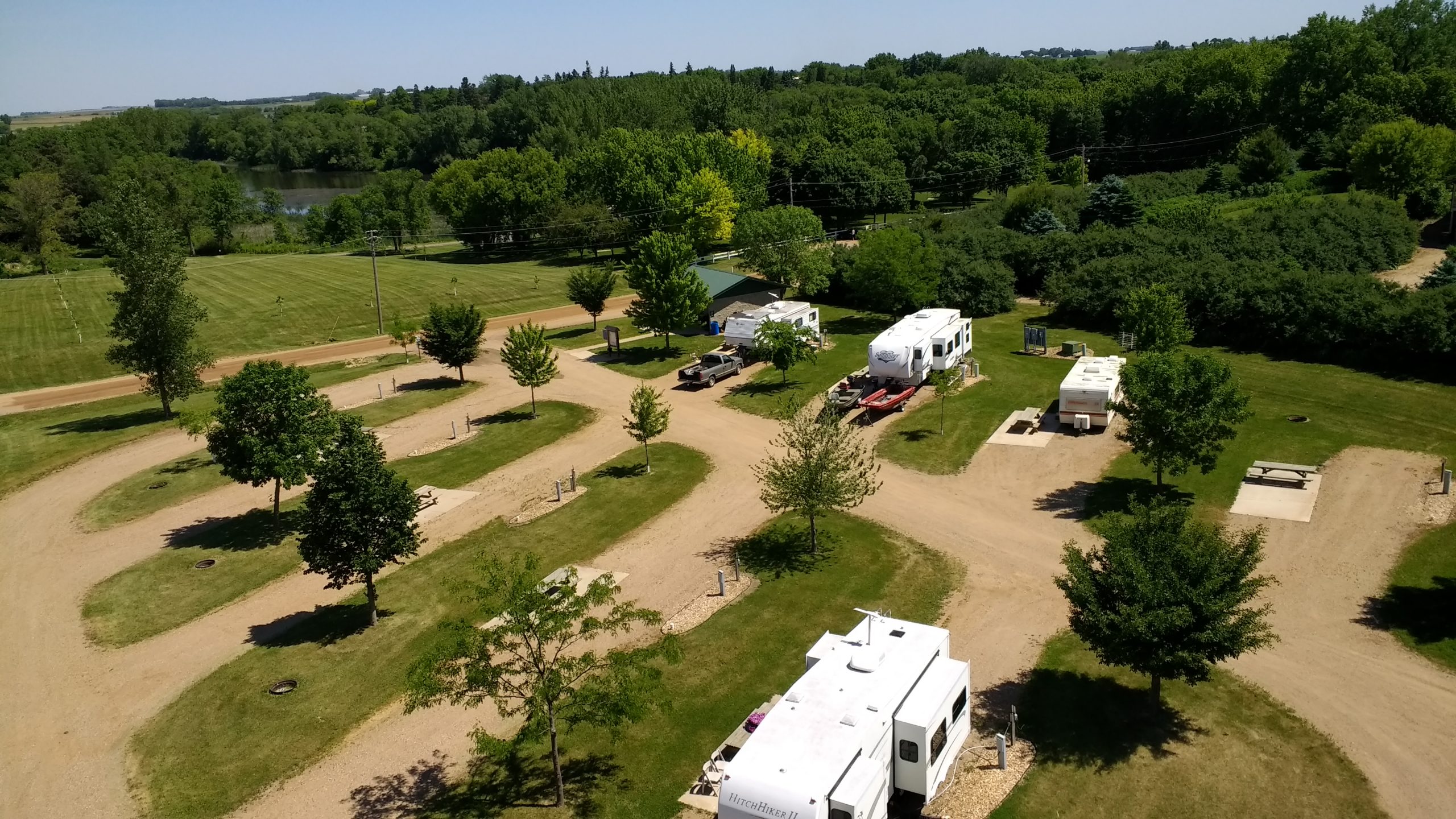This top-down image captures a serene summer campground enveloped by dense green foliage. The deep, vibrant greenery of the grass and trees paints a tranquil scene, emphasizing the lushness of the season. The campground features neatly graded dirt roads bisecting rectangular patches of green grass. Along these patches, there are four distinct trailer pull-throughs and several closely spaced parking areas, each accommodating one RV trailer. All four white RVs, each parked in a designated spot, are hooked up to water and electrical posts.

The foreground reveals a white RV nestled between two green plots, while a brown road extends from the center down to the bottom right of the image. Each green patch is flanked by small trees, contributing to the organized, yet cozy, layout. In the background, additional vehicles and smaller trees complement the setting, with a cluster of trees creating a verdant backdrop. Notably, picnic tables dot the area, suggesting spaces for communal gathering.

To the top left of the image, a truck appears to be loading items, and nearby, a shelter possibly housing public amenities is visible. A forest stretching across the horizon forms a natural boundary for the campground. Amidst the lush greenery and beneath a clear blue sky, the pastoral scene is accentuated by a power line running along the central road, connecting various utility posts and offering a subtle hint of modern convenience amid nature.